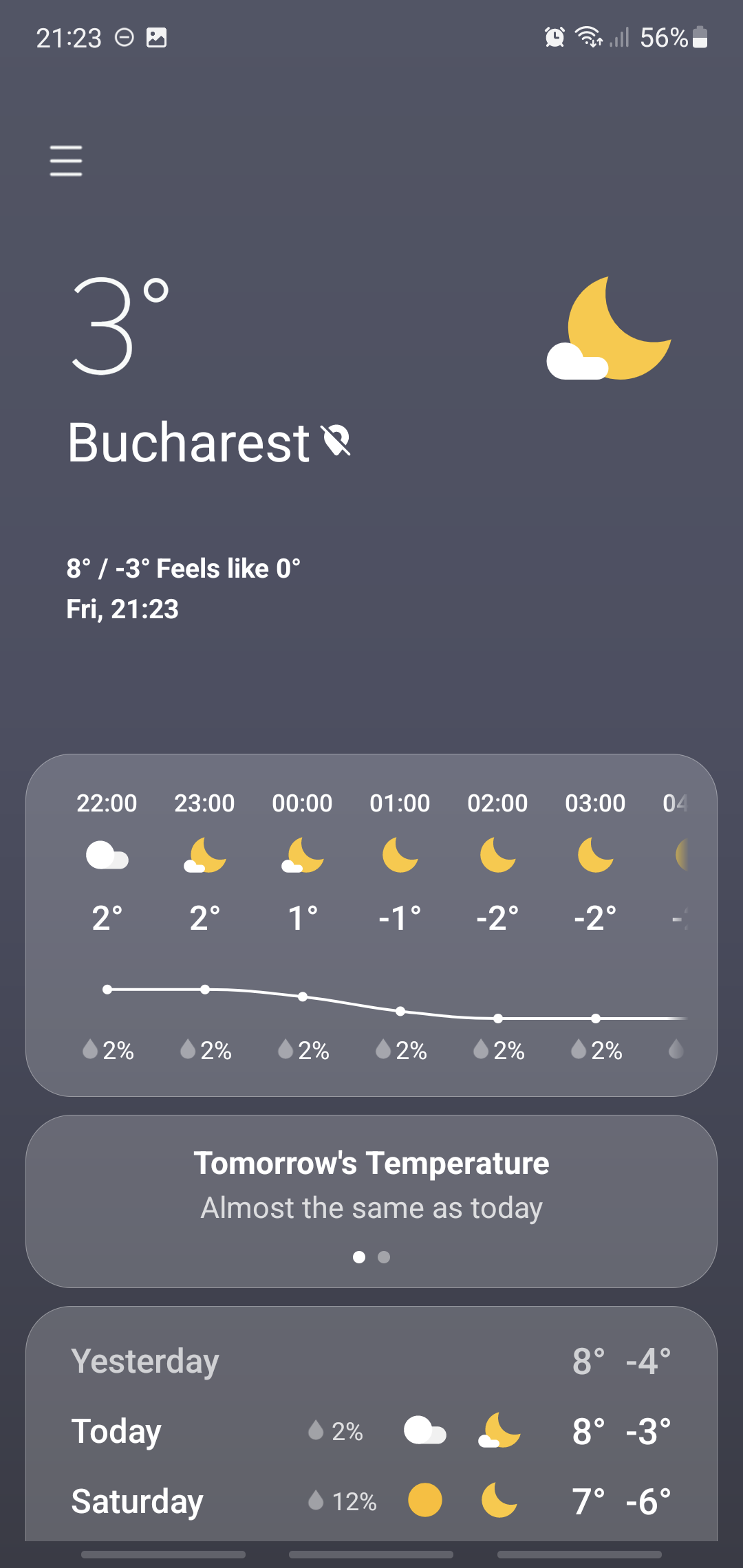In this image of a smartphone screen, the display features a sleek, grayish-black background. The phone's battery is at 56%, and the network connection is strong. The time is shown in military format as 21:33. There are three horizontal lines visible, indicating a menu or settings icon.

The weather app is open, showing the current conditions in Budapest. The temperature is 3°C, accompanied by an icon depicting a large moon and a smaller cloud. Additional weather information reveals that it feels like 0°C, with the actual temperatures being 8°C and -3°C (interpreted as 8°C feels like -3°C). 

It's Friday, and the date is January 23rd. The time is reiterated on the screen, and a detailed weather forecast is laid out. An arrow points to hourly updates, showing temperature changes and transitions from cloudy to partially sunny conditions. The icon, initially thought to be the moon, might be a partial sun due to the shift in weather conditions depicted throughout the day.

The app also compares today's weather with tomorrow's, which is expected to be similar. Two dots are displayed, one illuminated and one not, possibly indicating previous and upcoming days. The screen also provides weather statistics for yesterday, today, and Saturday, enabling a comprehensive understanding of the recent and upcoming weather patterns.